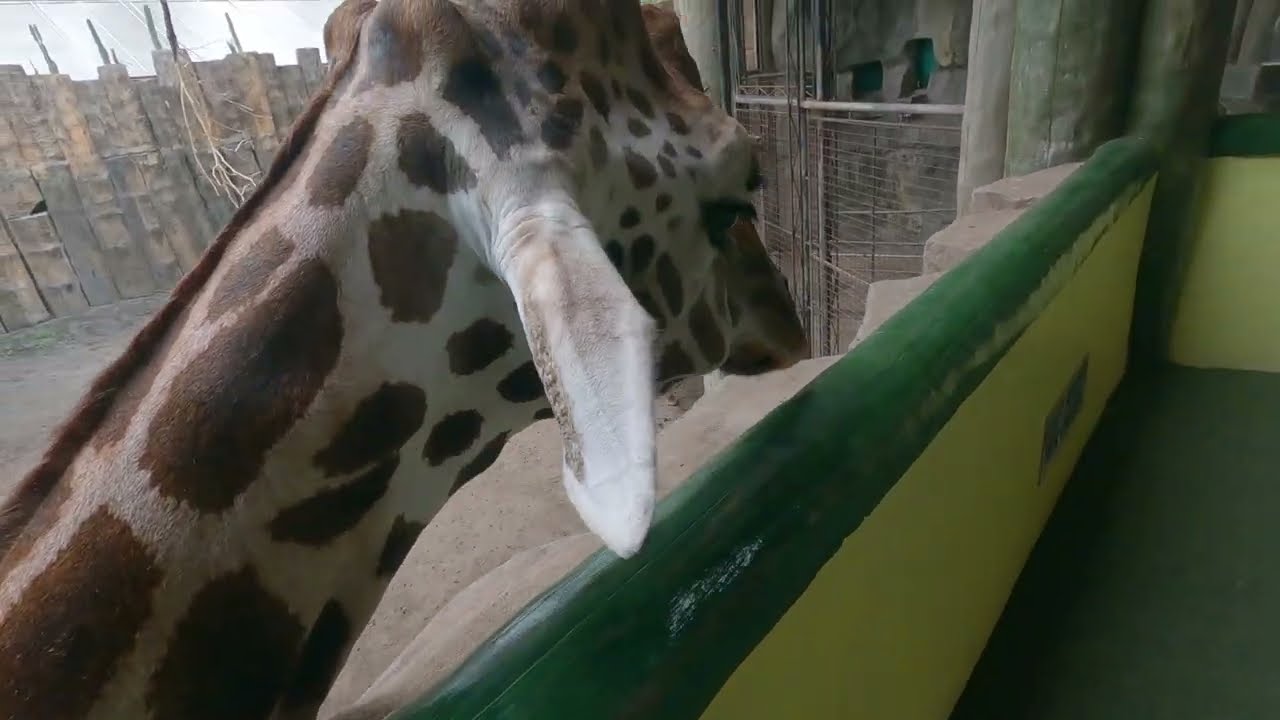This color photograph, taken in landscape orientation, features a close-up view of a giraffe's head and upper neck. The giraffe is looking away from the camera, and its distinctive markings and elongated neck are clearly visible. It appears to be peering over a barrier, presumed to be an observation deck at a wildlife facility. This barrier is primarily light lime green with a dark green border and stands about waist-high. The giraffe is positioned in an open-roofed area of its enclosure, with fake rock concrete walls surrounding it. In the background to the left, there is a driftwood plank fence adding a rustic touch to the enclosure, while other fences and wood supports can be seen to the right. The ground of the enclosure is a sandy beige color, emphasizing the naturalistic setting.